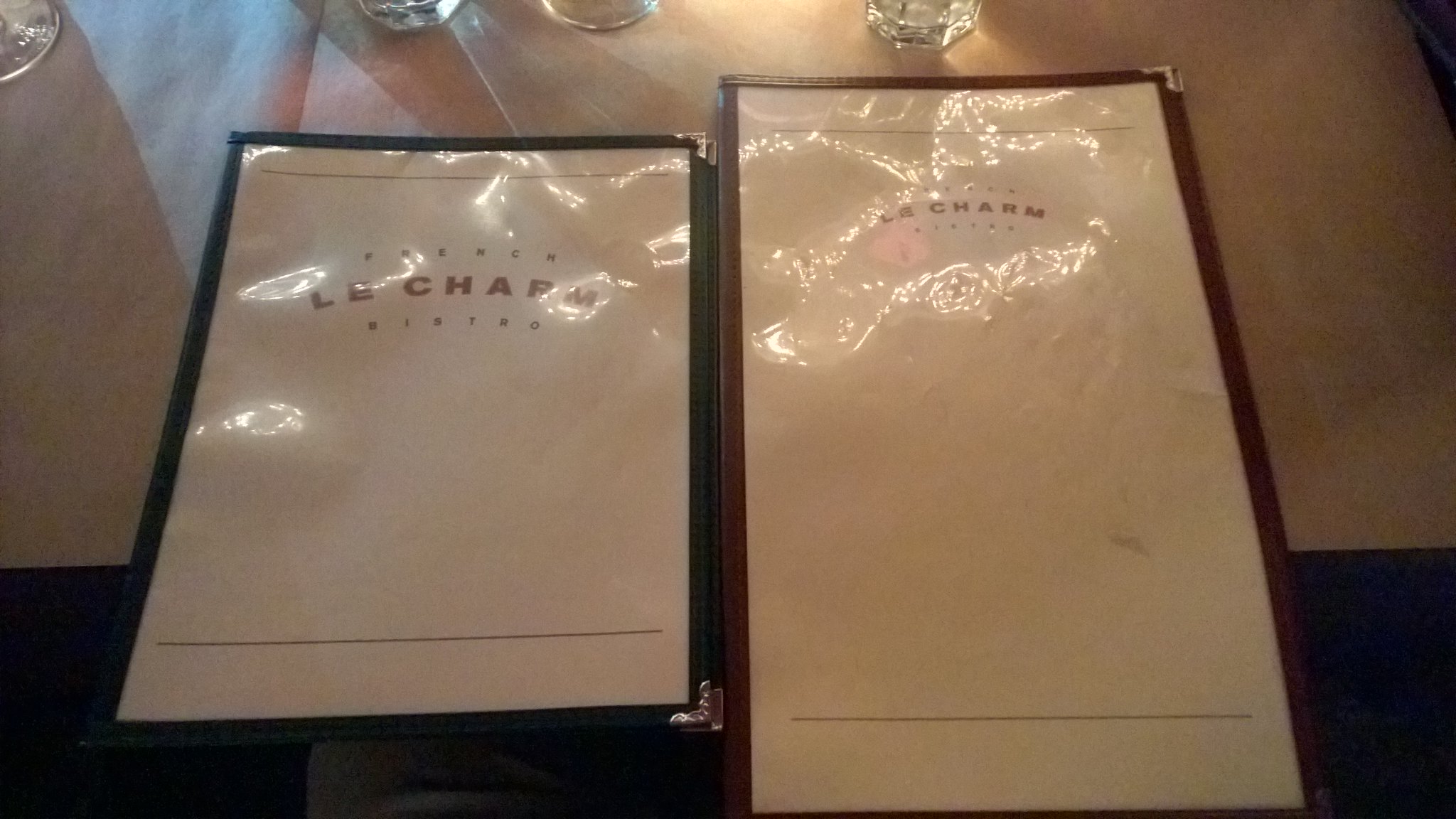In the photograph, we see a dining table at a restaurant, adorned with what appears to be vintage or higher-end menus. These two menus are positioned side by side, each enclosed in vinyl with small metal corner tips. The vinyl edge on the left menu is black, and despite originally housing white paper, the paper now appears grayish-pink due to the lighting or age. This menu is slightly shorter and bears the inscription "French Le Charme" at the top, with "Bistro" underneath, separated by a thin horizontal line. Light from above reflects off its surface, making the text challenging to read.

Adjacent, the second menu is larger and features a similar design, bound in dark burgundy vinyl. Though the text is partially obscured by glare, it can be inferred it also reads "French Le Charme" at the top and "Bistro" at the bottom. Both menus reflect overhead light, casting a bright sheen over their surfaces.

The table itself appears to be draped with a tablecloth. Four glasses are arranged on the table, possibly varying in type. Two of them are likely water glasses, characterized by their heavier, chunkier build. The other two glasses seem to have circular bases, which hints they could be stemmed glasses like wine glasses, although their stems aren’t clearly visible in the photograph.